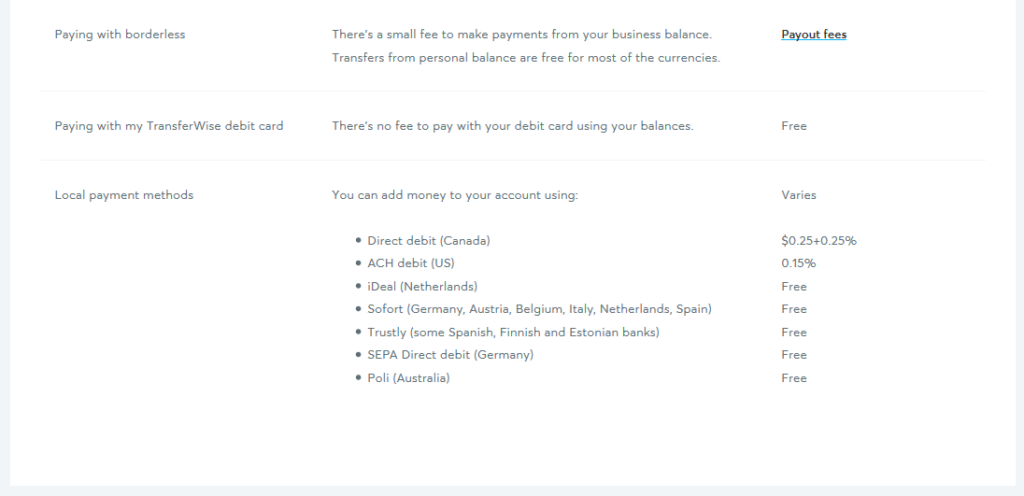The image features a white background with a gray border that partially frames it—vertically on the left and right sides, and horizontally at the bottom, giving the impression of a zoomed-in view. The inner background is light gray and divided into three distinct columns filled with text.

Starting from the left column, the first line reads in gray text: "Paying with borderless." Below it, another line states: "Paying with my TransferWise debit card." Further down, it reads: "Local payment methods."

The middle column contains a detailed explanation about fees: "There's a small fee to make payments from your business balance. Transfers from a personal balance are free for most currencies." It also adds: "There's no fee to pay when your debit card uses your balance."

This section continues with information on adding money to your account through various methods, formatted with bullet points:
1. Direct debit (Canada)
2. ACH debit (U.S.)
3. iDEAL (Netherlands)
4. SOFORT (Germany, Austria, Belgium, Italy, Netherlands, Spain)
5. Trustly (Finnish, Estonian, Spanish banks)
6. SEPA direct debit (Germany)
7. POLi (Australia)

Towards the bottom, a line underlined in blue states: "Payout fees". This is followed by several fee structures:
1. Free
2. Specific rates
- $0.25 + 0.25%
- 0.15%
- Free, free, free, free, free

This caption elaborately describes the layout and textual content visible in the image, offering clear details about the listed payment methods, associated fees, and international applicability of the services described.